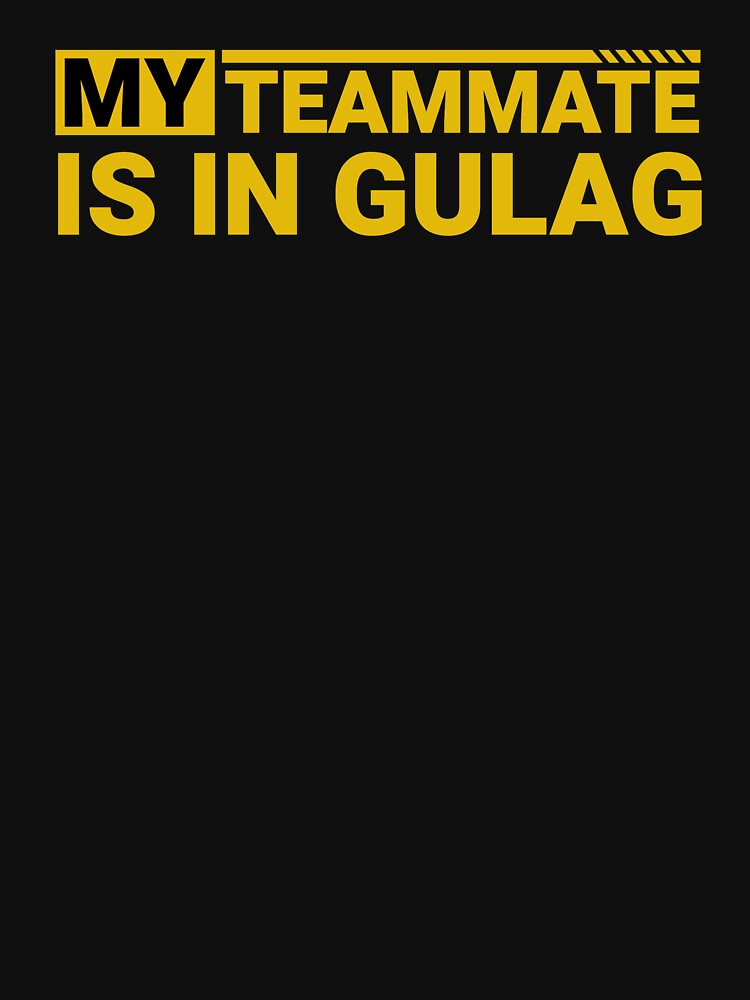The image features a predominantly dark background with text positioned in the upper one-third of the frame. The text, arranged in block letters and entirely capitalized, reads "MY TEAMMATE IS IN GULAG." The word "MY" is written in black font within a yellow rectangle, creating a strong contrast against the dark backdrop. Below "MY," the word "TEAMMATE" is displayed in yellow font, accompanied by a horizontal yellow line above it. This line extends from the beginning to the end of the word "TEAMMATE" and features six diagonal strokes at the far right end, which create gaps that reveal the dark background beneath. The remaining words, "IS IN GULAG," are also in yellow font and situated on the second line of the text. The overall composition conveys a stark and attention-grabbing message with no additional elements or decorations, making the text the focal point of the image.